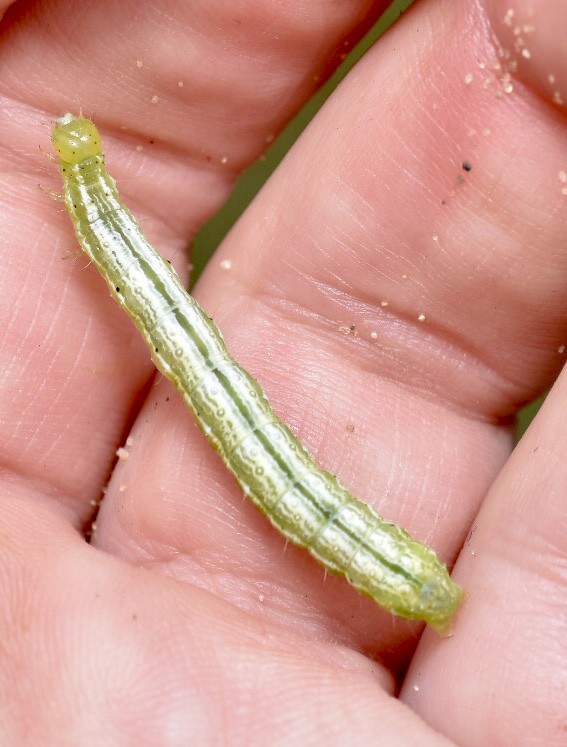This full-color, daytime photograph captures a meticulously posed nature shot outdoors. At the forefront of the image are three fingers of a Caucasian person, each dusted with grains of sand, suggesting the scene might be in a wilderness area or garden. Resting in the center of the person's hand is a long, primarily green caterpillar with distinct white stripes along its back. The caterpillar's head is a large, bulbous olive-green sphere adorned with some black specks and a touch of white. Tiny, hairy projections can be seen at the bottom of the caterpillar, which assist in its movement. The soft green blur in the background hints at vegetation, adding to the natural setting of the photograph. The colors in the image include tan, pink, green, white, and black, enhancing the detailed and vivid portrayal of this tranquil moment in nature.